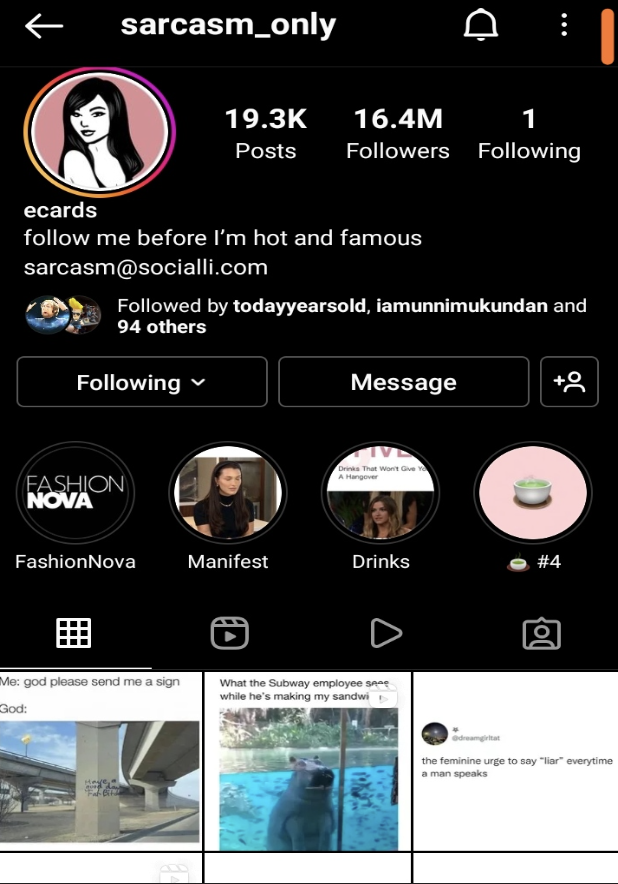Screenshot of the "Sarcasm Only" Web Page on an App:

The screenshot showcases a web page from the "Sarcasm Only" app. At the top, there's an arrow pointing to the left labeled "sarcasm_only." To the right of that, icons for alerts (a bell) and more options (three vertical dots) are visible. Below these icons is an orange bar.

Beneath the orange bar, there is a round profile picture of a cartoon woman shown from the chest up. Accompanying text indicates that this user has 19.3 thousand posts, 16.4 million followers, and is following one person. The profile title reads "e-cards" with the bio, "Follow me before I’m hot and famous - sarcasm." The user handle is @socialeye.com.

The account is followed by notable users such as "today years old," "I am unnimbocantant," and 94 others. Below this is a row of buttons labeled "Following," "Message," and an "Add" button. 

Further down, the page suggests other popular users on the app such as "Fashion Nova," "Manifest," "Drinks," and "Number Four." 

Finally, there are four distinct icons, followed by a series of posts. The posts include: 

1. A meme stating, "Me: God please send me a sign" with an accompanying image.
2. "What the subway employees see when making your sandwich."
3. "The feminine urge to say 'liar' every time a man speaks."

This detailed layout highlights the interactive and humorous content available on the "Sarcasm Only" app.